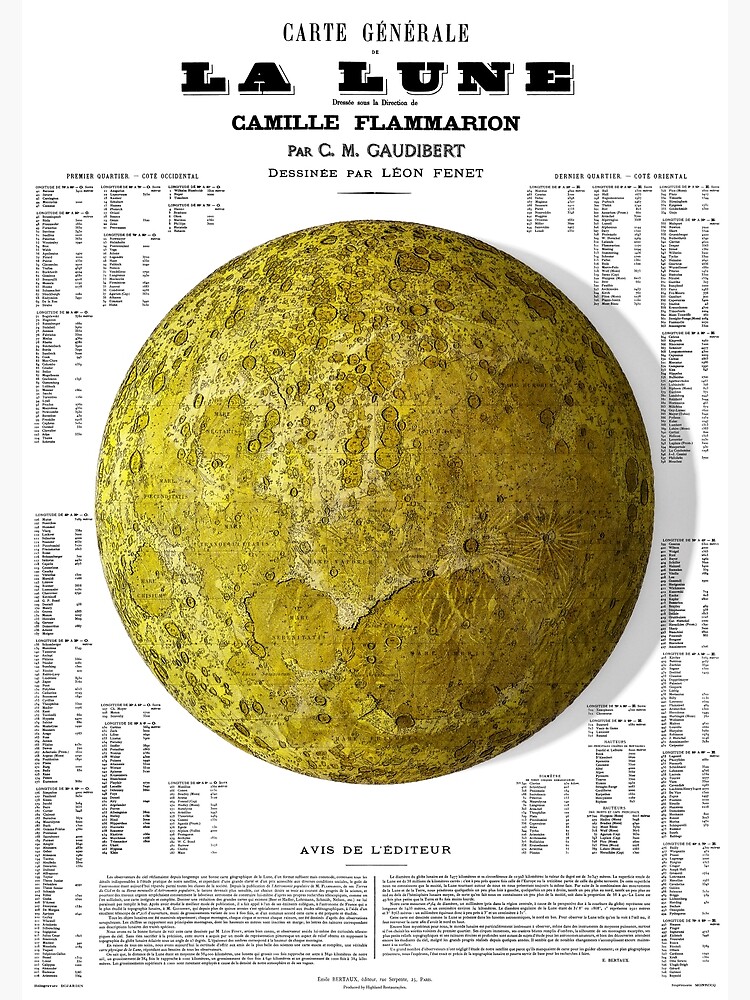The image shows an illustrated globe, likely of the moon, given the prominent text. At the top of the image, in black font, "Carte Générale" is clearly visible, followed by "LA LUNE" in larger, bold letters, suggesting a detailed map of the moon. Underneath "LA LUNE," the name "Camille Flammarion" is printed. The depiction of the moon is spherical, complete with recognizable craters, and has a greenish-yellow hue with darker brown areas, adding to the uncertainty of its identity. Surrounding the globe is a significant amount of very small text in black font on a white background, providing further explanation and details, although it is mostly unreadable. Additionally, there is some noticeable shadowing around the right side of the moon, giving it a more three-dimensional appearance.